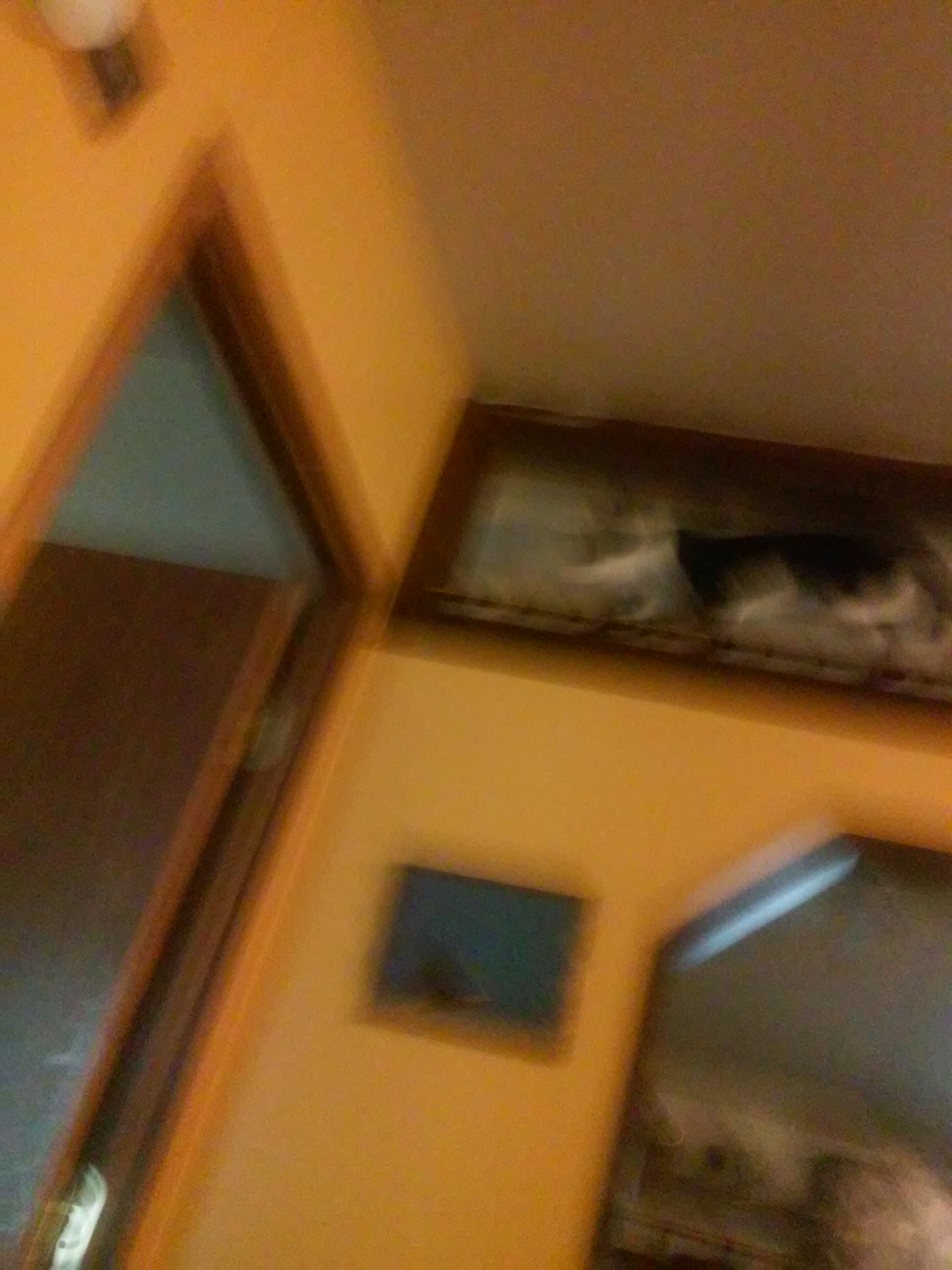This color photograph is noticeably blurry, creating a sense of disorientation. The perspective suggests it was taken from a low angle, either by someone lying down or looking upwards. The room features striking orange walls, adding a warm, vivid backdrop to the scene. On the left side, an open doorway is visible, hinting at an adjoining room. Dominating the center, albeit diagonally, is a long, framed piece of art, though its details are indistinguishable due to the lack of focus. Beneath it hangs a smaller piece of art, equally obscured and nondescript. In the bottom right corner of the photograph, part of a mirror is captured, reflecting more of the blurred surroundings. Overall, the image, with its abstract portrayal of an orange-hued room adorned with unclear artworks and a mirror, invites curiosity but leaves much to the imagination due to the pervasive blurriness.